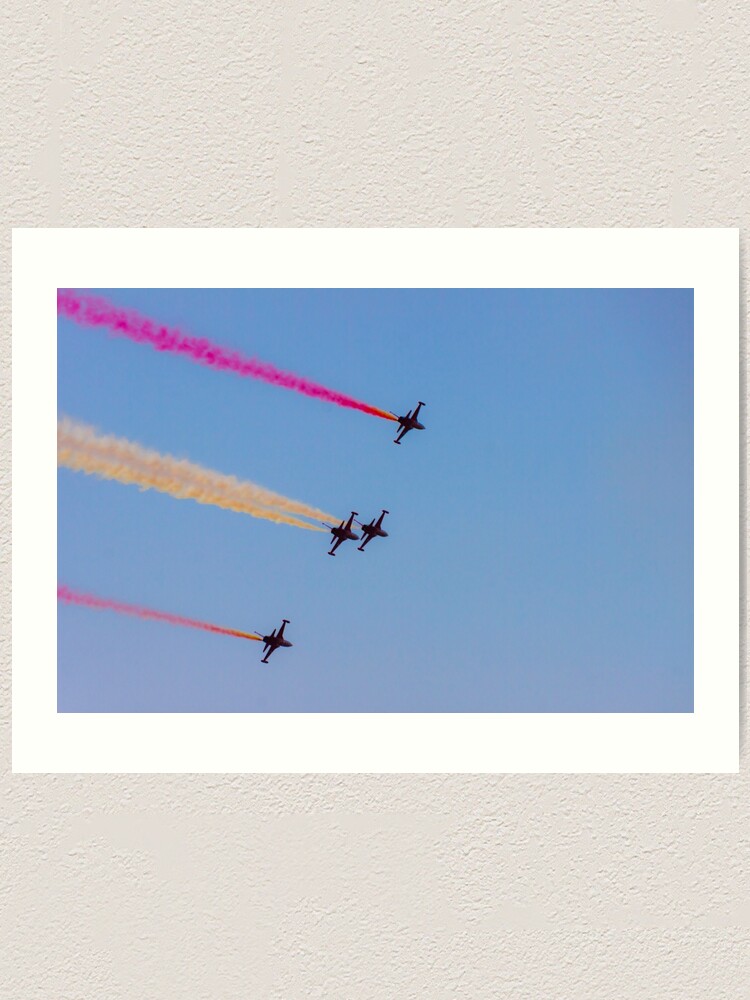Displayed against a textured, cream-colored wall, this photograph is framed in white and showcases a thrilling aerial demonstration. Set against a bright, clear blue sky with a slight gray haze near the bottom, four jets are captured flying in precise formation. The two central jets are extremely close, appearing as though one is flying directly above the other, and both trail streams of white, gold, or light peach-colored smoke. Flanking these central jets are aircraft on either side; the jet on the far left releases a trail of orange to reddish-pink smoke, while the jet on the far right leaves a distinctive bright red plume. This captivating image, likely taken during an air show on a sunny day, highlights the precision and artistry of the aerial maneuvers.